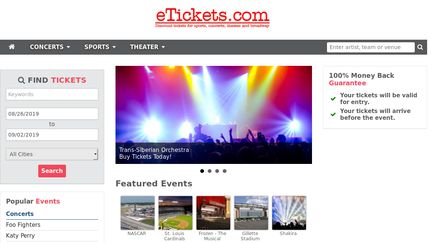This image showcases a detailed web page layout for e-tickets.com. At the very top, "e-tickets.com" is prominently displayed in red against a clean white background. A black navigation bar spans across the upper section, featuring a home icon on the far left, followed by white text links for "Concert," "Sports," and "Theater" with associated drop-down menus. On the far right of this bar, there's a search function allowing users to look up artists, teams, or venues.

On the left-hand side, a gray box titled "Find Tickets" offers search options by keywords, dates, and cities, including a bright red search button. Below this box, in the bottom left corner, a list of popular events is displayed, highlighting concerts such as those by the Foo Fighters and Katy Perry. "Events" is marked in red, while "Concerts" is in blue.

Central to the page, an eye-catching image features a vibrant, multi-laser light concert scene advertising the Trans-Siberian Orchestra, urging visitors to buy tickets with a note that the orchestra has a strong metal influence.

Further down, the "Featured Events" section lists major events, including NASCAR and the St. Louis Cardinals, with Shakira's upcoming performance also noted.

On the right-hand side, a small white box reassures customers with a "100% Money Back Guarantee," emphasizing in red text. The box includes checkmarks next to two assurances: "Your tickets will be valid for entry" and "Your tickets will arrive before the event."

Overall, this comprehensive and user-friendly web page offers various options for purchasing tickets, presenting a viable alternative to other major ticketing sites.